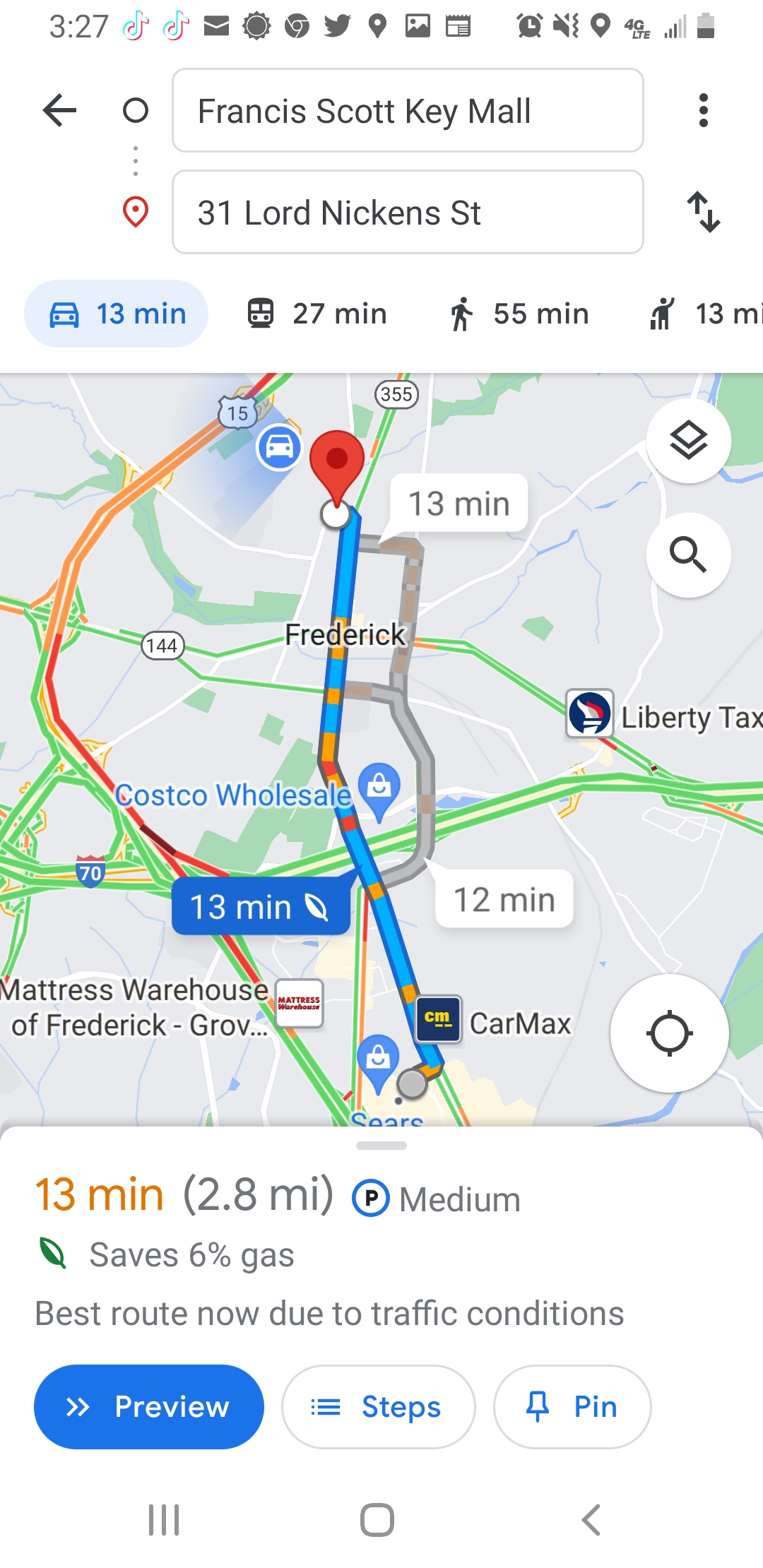This detailed screenshot of a phone screen captures a Google Maps navigation session. The primary focus is the route from Francis Scott Key Mall to 31 Lord Nickens Street. A blue line indicates the path, which is predicted to take 13 minutes covering a distance of 2.8 miles. Traffic conditions are affecting the journey slightly, but the current route is optimized, saving 6% on gas usage. At the bottom of the navigation screen, several buttons are visible: "Preview," "Steps," and "Pin." Additionally, the phone's menu navigation bar is visible at the bottom of the screen.